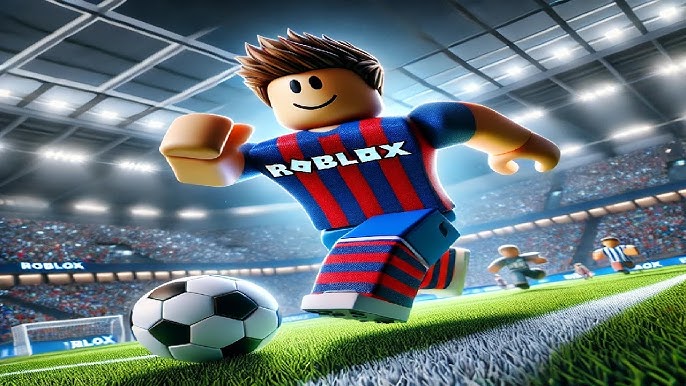The image showcases a digitally enhanced logo for Roblox Soccer set against a dark blue background, which transitions through lighter shades of blue and culminates in a luminous teal or aqua hue at the center. The logo itself is hexagonal, resembling a diamond-like, vertical crest with elongated sides and shorter top and bottom edges that make it slightly pointed. Encircling the logo is a light silver outer rim that emits a glowing effect extending into the background. 

At the heart of the crest is a prominently featured soccer ball adorned with classic black and white hexagons, subtly illuminated by a greenish glow at its base. Below the soccer ball, the word "ROBLOX" is displayed in a large, futuristic, and chunky all-caps font, with each letter appearing squared and thick. Notably, the first "O" is tilted diagonally to the right, leaning slightly against the adjacent "B". Underneath "ROBLOX", the word "SOCCER" is printed in smaller, all-caps white font, less blocky than the one above. The entire logo is suffused with a radiant greenish glow projecting from the crest, enhancing its vibrant and eye-catching appearance.